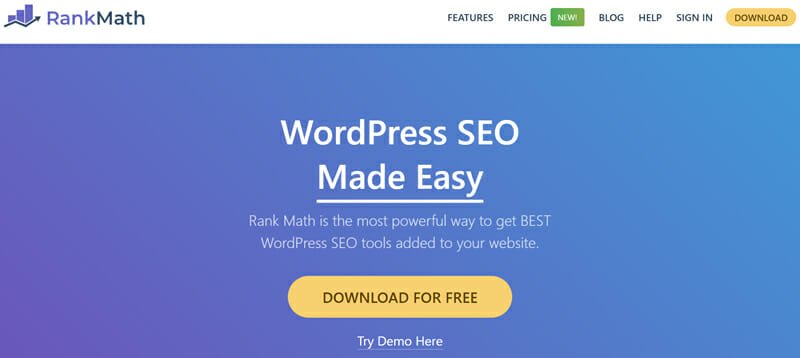Screenshot Description:

The screenshot depicts a webpage from Rank Math. At the top, a white horizontal banner spans the width of the page. In the upper left-hand corner of this banner, there's a graph-like icon characterized by a zig-zag arrow pointing upwards to the right, with three rectangular boxes positioned atop the arrow. Adjacent to the icon, the text "Rank Math" is displayed, where "Rank" is in blue and "Math" in black. 

On the right side of the banner is a menu featuring several options: Features, Pricing (with a green 'new' icon next to it), Blog, Help, Sign In, and Download. The Download option is highlighted with a wide, yellow, oval shape.

Below the white banner, the background transitions from a darker blue, almost purple hue on the left, to a lighter blue on the right. Centrally positioned on this background is the text "WordPress SEO Made Easy," with "Made Easy" underlined. Beneath this headline, a subheading explains that "Rank Math is the most powerful way to get the best WordPress SEO tools added to your website."

At the bottom center of the page, a prominent yellow oval button with the text "Download for Free" is displayed. Below this button, there is a smaller text link that reads "Try Demo Here."